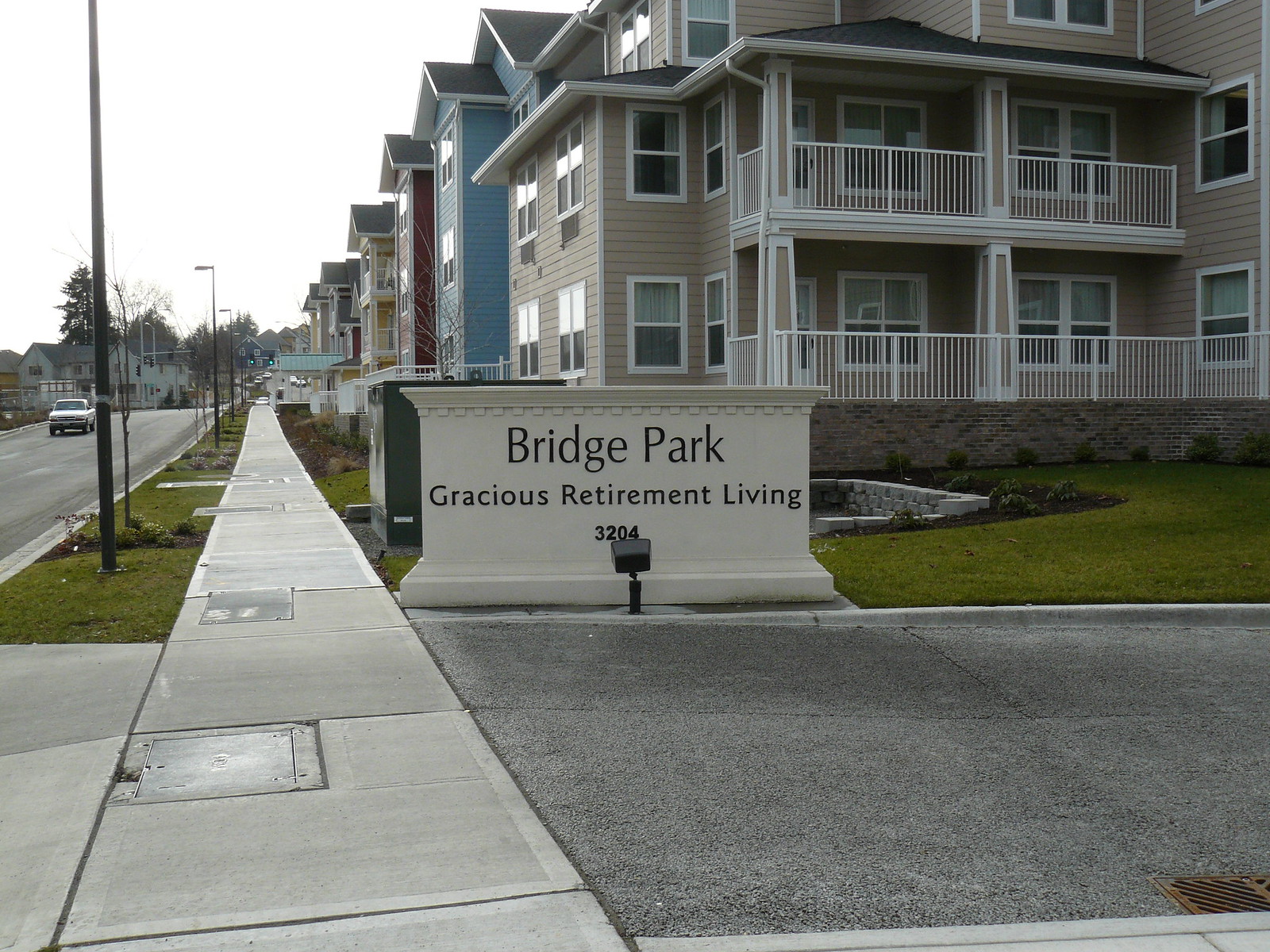This photograph, taken from the perspective of a sidewalk during daylight, captures the entrance of a retirement community named Bridge Park Gracious Retirement Living at 3204. A prominent white stone sign with black lettering stands in the foreground, slightly to the right, with a decorative crown trim molding on top. In front of the sign, there is a black spotlight on the ground, currently off due to the daylight sky. The scene includes a paved driveway entrance immediately beyond the sign and expanses into a series of three-story townhouses with white windows, porches, and balconies. The buildings are sequentially colored in beige, light blue, maroon, and mustard gold. To the left of the image is a dark gray concrete sidewalk parallel to a street with a white vehicle visible. The grass in front of the buildings is well-maintained in green, contrasting with the mixed hues of the townhouses and the neutral tones of the pavement. In the background, additional buildings can be seen under a light sky, indicating a typical day scene.